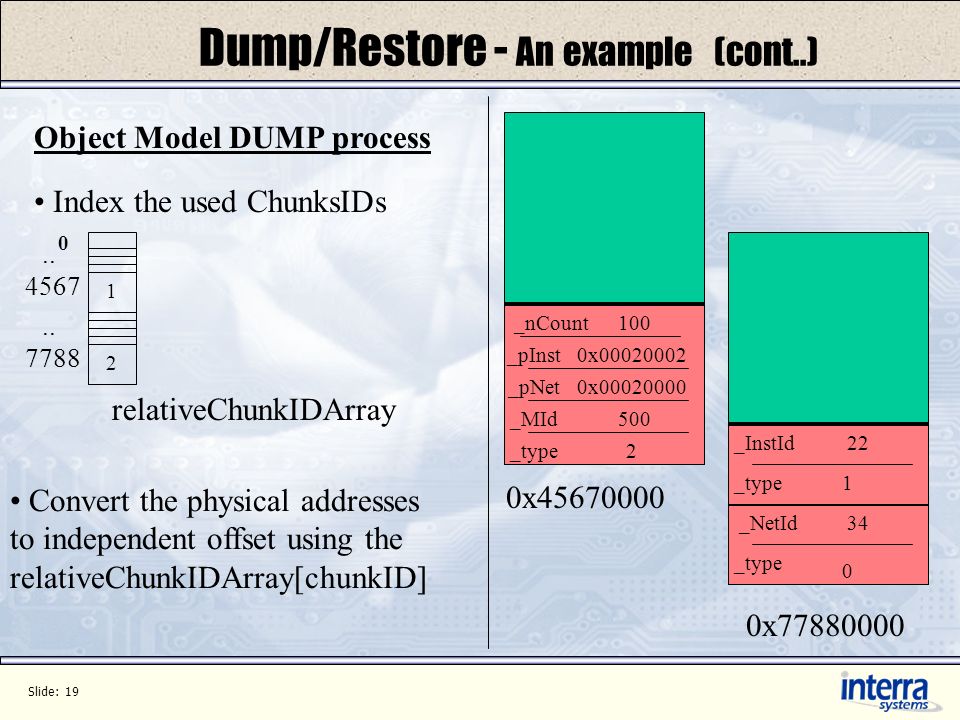This image is a detailed rectangular chart used in a presentation. Measuring approximately six inches wide and four to five inches tall, the chart features a header at the top with a brownish-gray stone coloring and thin black pinstripes outlining it. The header text, in bold black print, reads: "dump/restore - an example (CONT...)". Below the header, the chart is divided into a left and right panel against a light bluish-gray background with an indiscernible design overlay.

The left panel details the "Object Model DUMP Process" in underlined black print, with "DUMP" in all capital letters. It lists several steps: a bullet point stating "Index the used chunks IDs," followed by a visual bar graph with numbers 0, 4, 5, 6, 7, and 7, 7, 8, 8, and labeled "Relative Chunk ID Array". Another bullet point below instructs to "convert the physical addresses to independent offset using the relative chunk ID array (chunk ID)".

The right panel displays two sets of rectangles, each divided into a green top half and a red bottom half. The left rectangle's red bottom lists details such as "END COUNT 100", "PINST 0x0002000002", "PNET 0x2000000", and "MID 500 TYPE 2". Below these, it displays "0x45670000". The right rectangle’s red bottom shows "INST ID 22 TYPE 1" and "NET ID 34 TYPE 0", followed by "0x77880000" in black print.

At the bottom of the chart, there is a light brown footer. The left side of the footer states "Slide 19" in black print, and the right side, in blue print, reads "Intera Systems".